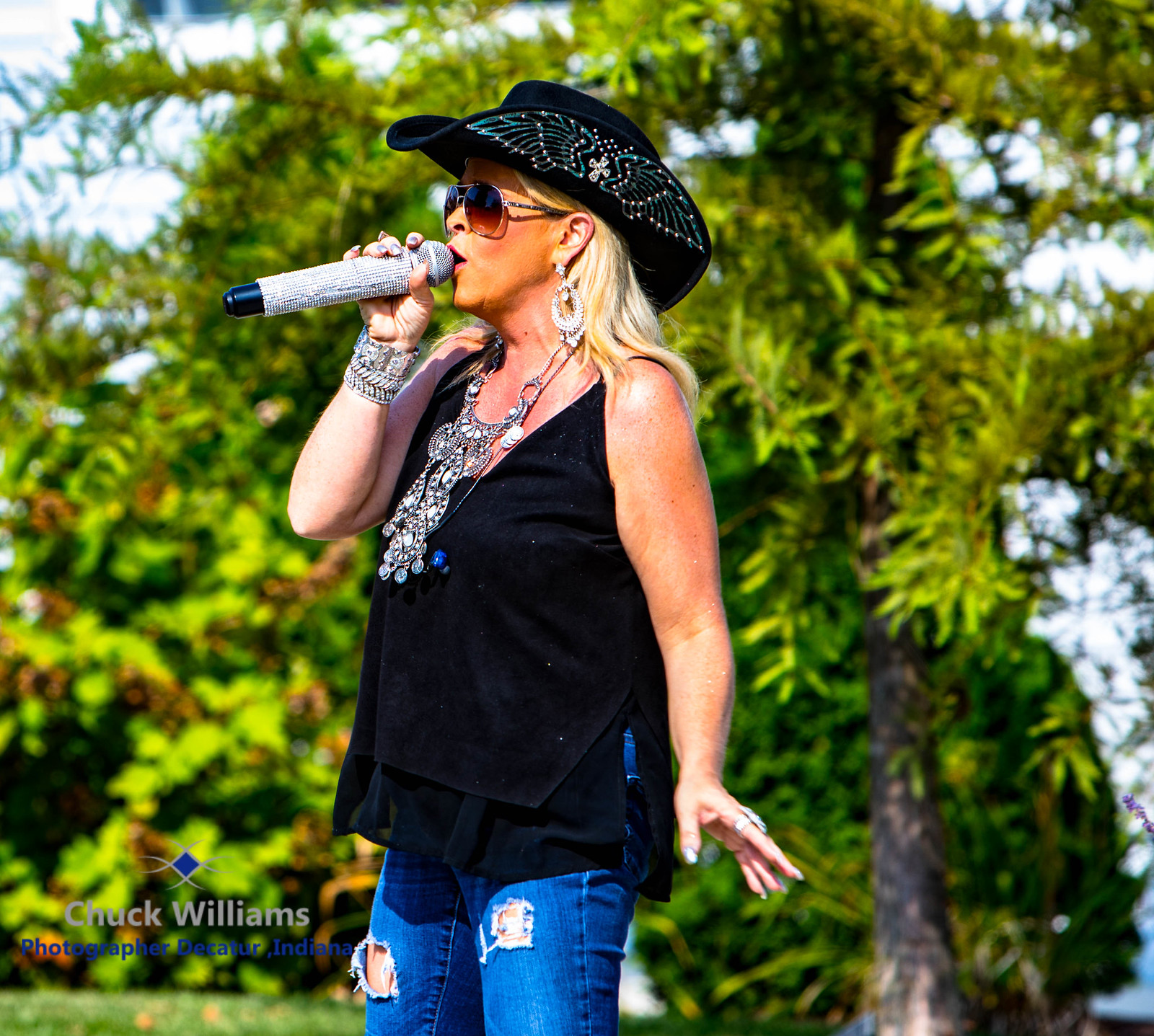In this image, a middle-aged, tanned woman with blonde hair stands as the main focus, centrally positioned and presumably singing into a wireless microphone. The microphone is adorned with dazzling decorations except for its black tip. She is attired in a loose black tank top and blue jeans with distressed and ripped areas in the front. Accentuating her outfit, she wears a cowboy hat embroidered with silver wings and a flower in the center. The woman's jewelry includes a necklace with silver bangles and three silver bangle bracelets on her wrist. Sunglasses shield her eyes as she stands against a slightly blurred outdoor backdrop featuring a field of grass, leaves, and a mix of trees and bushes. The setting suggests a daytime concert, with the colors comprising shades of green, light blue, black, silver, white, and gray. A watermark is visible in the bottom left corner, reading "Chuck Williams, photographer, Decatur, Indiana" in silver and blue text.